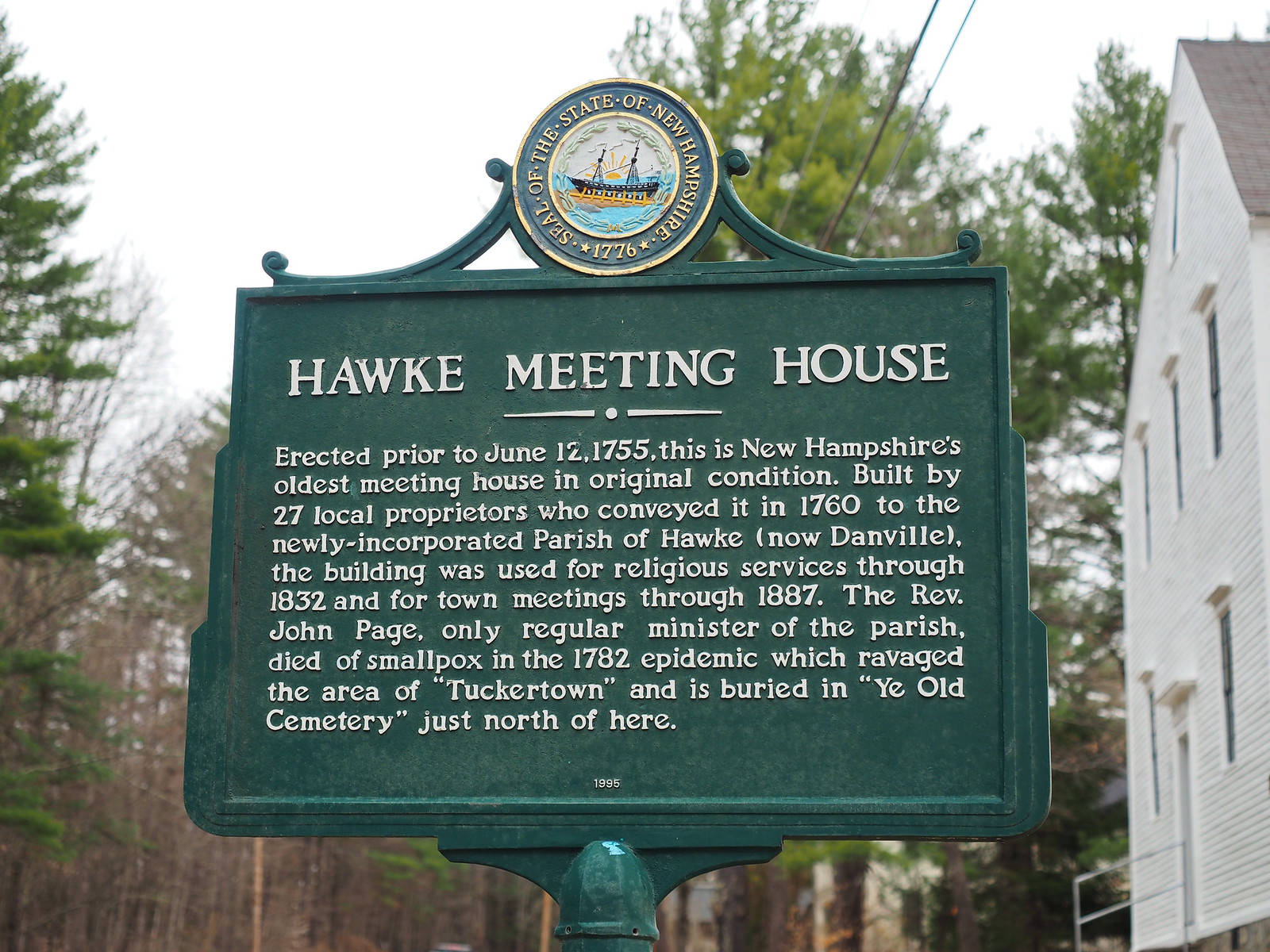This photograph captures a green metal sign prominently displaying historical information. At the top, a round emblem features the words "State of New Hampshire, 1776," encircling an intricate painting or engraving of a ship. Below the emblem, the sign is titled "Hawk Meeting House," followed by a detailed description of the meeting house itself. The text on the sign is rendered entirely in white, using a font that resembles old typewriter text, adding a vintage feel. The sign is situated outdoors, positioned in front of a white building. The background is lush with tall, green trees, enhancing the rustic and historical ambiance of the scene.